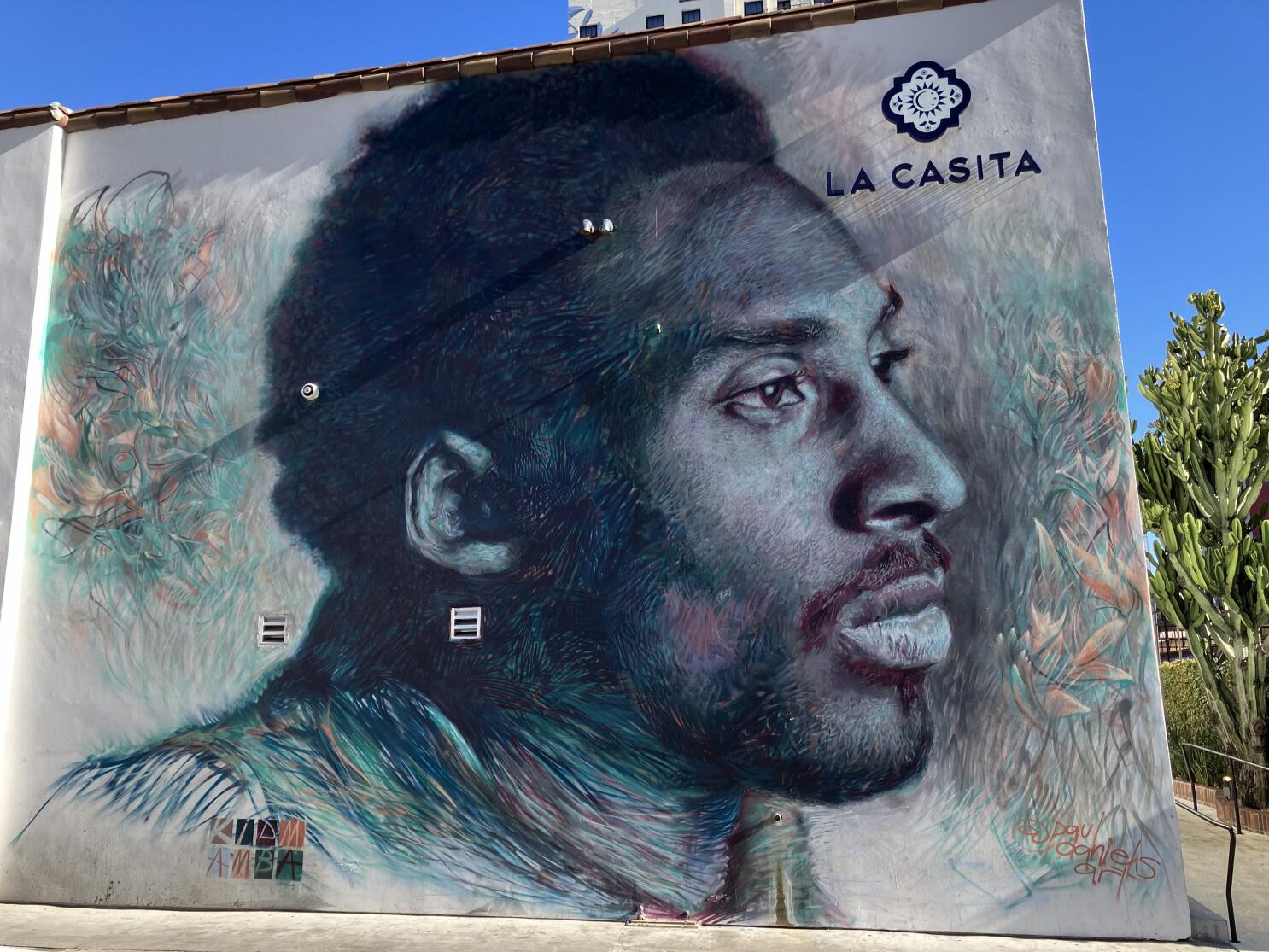The image is a square-shaped wall mural of Kobe Bryant, capturing him in a somber side profile from his shoulders to the top of his head. Kobe's dark hair, mustache, and thin beard are meticulously rendered, emphasizing his full lips and long eyelashes. The mural employs a painterly effect around his neck and shoulders, transitioning into a more realistic black and white tone for his face and head. Above the portrait, a Moroccan-shaped white emblem with a burst design contains black text reading "La Casita." The wall features handwritten block letters on the bottom left spelling "K L A M A M B A" and a signature by "Daniels Art," though the full text is mostly illegible. Behind the mural, a clear blue sky can be seen along with a brown-tiled roof edge. The right side of the wall reveals hints of a green tree and a rail in front, contributing to the background landscape.